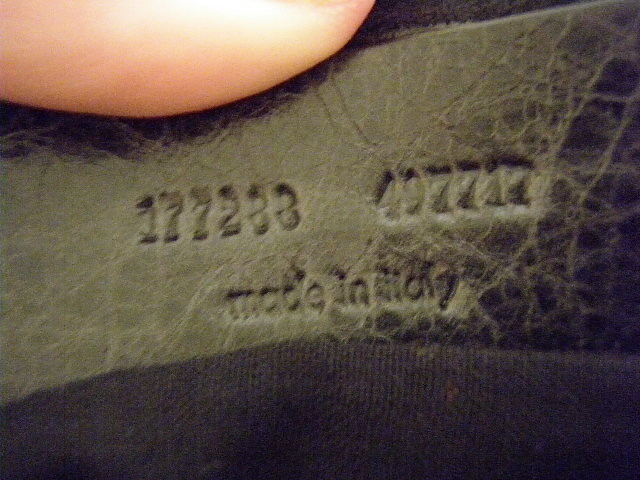A detailed caption for the image could be:

"This finely crafted belt, made in Italy, showcases a unique blend of elegance and ruggedness. The surface features the numbers '177233' and '497712' subtly pressed into the material, while the 'Made in Italy' inscription is etched in a slightly worn, yet still readable, fashion. The leather is characterized by its pronounced wrinkles and deep crack marks, giving it a distinctive vintage appeal. The edges are reinforced with a contrasting black fabric, providing a striking frame for the belt’s weathered appearance. The reverse side presents a lighter black hue, adding to the overall sophisticated yet rugged design."